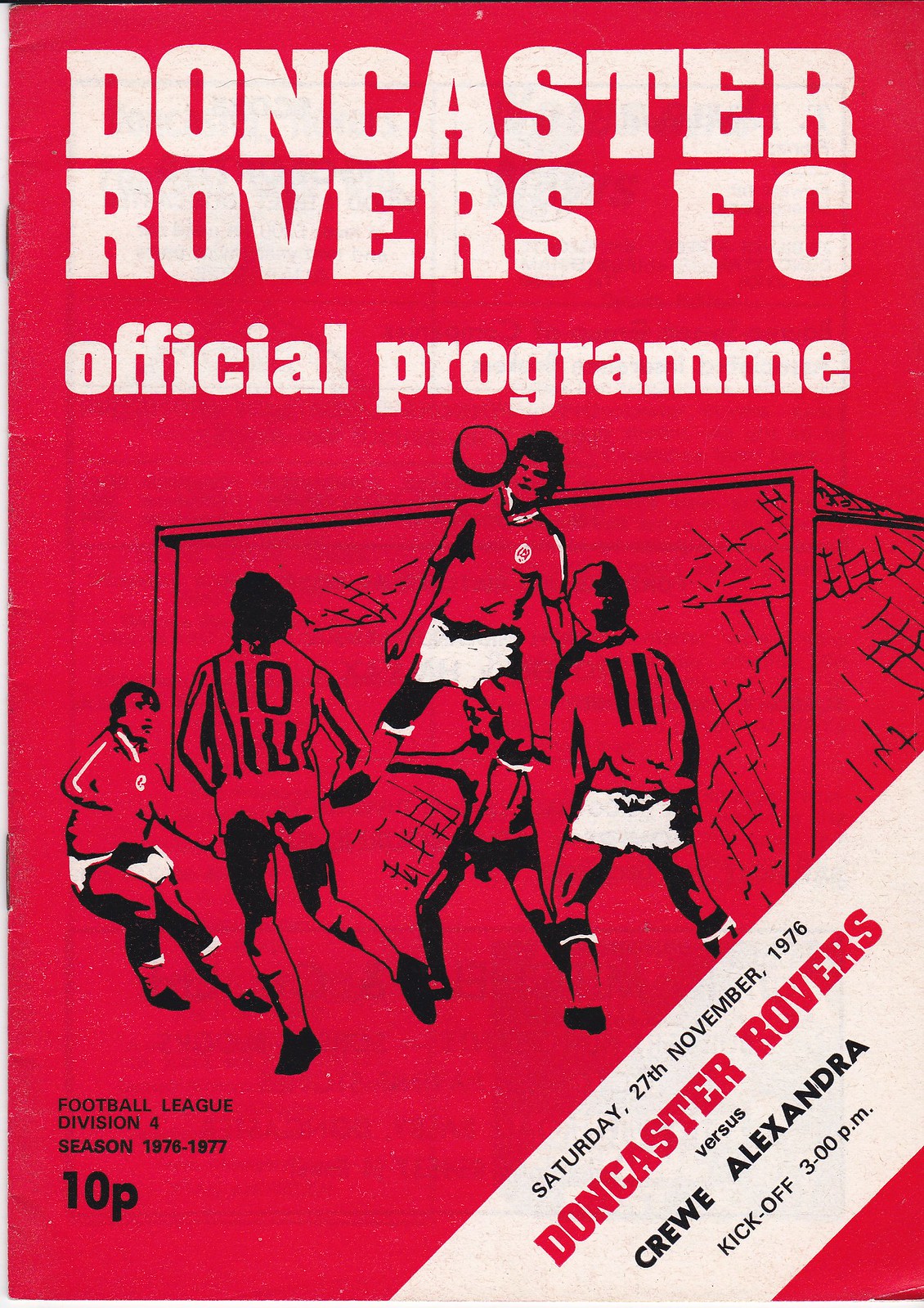The image is of a red-colored Official Program (spelled "Programme") for Doncaster Rovers FC. At the top, "Doncaster Rovers FC" is prominently displayed in white. Below that, there's a black and white graphic depicting soccer players in action, with one player deflecting a ball with his head in front of a goal. Referees and multiple teams are also visible within the graphic. On the bottom left, it states "Football League Division Four Season 1976-1977" and the price "10P" (10 pence), all in black. On the bottom right, within a white angled band, it reads "Saturday, 27th November 1976, Doncaster Rovers vs. Crewe Alexandra, Kickoff 3 p.m." The program encapsulates the match details and date in a visually striking red and white color scheme.